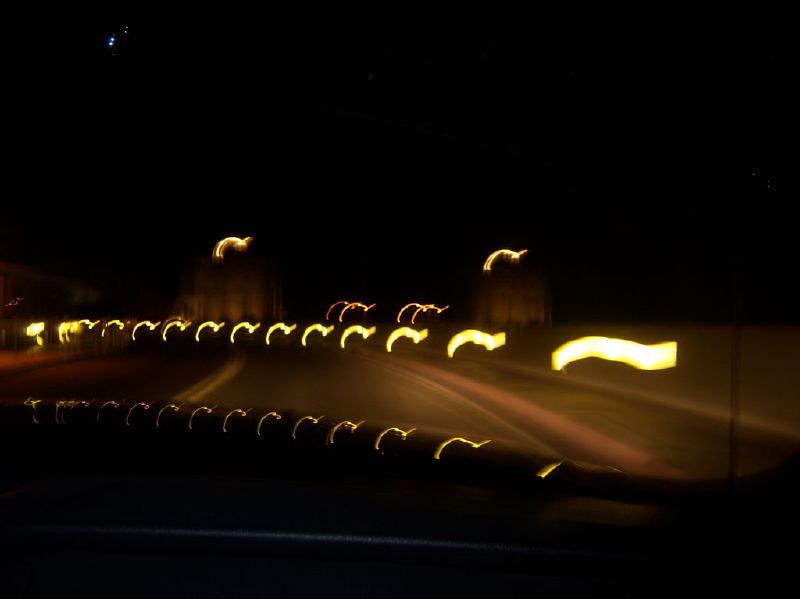This photograph appears to have been taken from a moving car, capturing a dynamic scene with significant motion blur. The top edge of the dashboard and the car's hood are visible at the bottom of the frame, grounding the viewer in the vehicle. The road stretches ahead, with a double yellow line positioned to the left, indicating that the car is traveling on the right side of the road. The surroundings are blurred, but two buildings can be made out on the horizon. One building stands closer to the left edge of the road, while the other is situated slightly farther back to the right. A hint of a sidewalk follows the road's curve, and indistinct streaks of light, possibly reflections from barriers or streetlights, add to the sense of motion. The overall impression is one of speed and movement, with the scene rendered in a dreamlike, almost abstract form due to the blur.